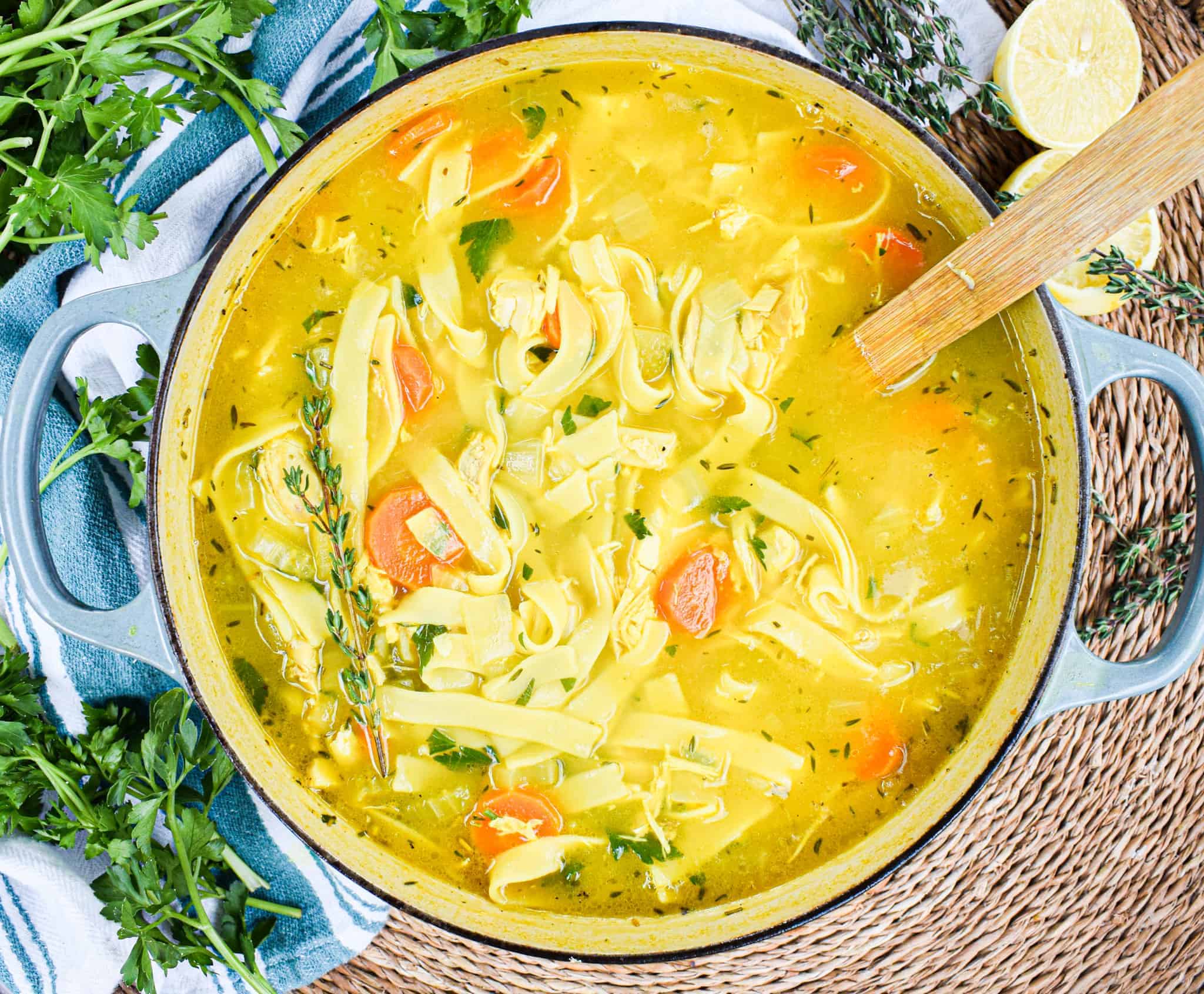This overhead photograph captures a vibrant pot of homemade chicken noodle soup set on a straw placemat. The pot, prominently occupying the center of the image, features blue handles positioned to the left and right. A wooden spoon extends from the soup, its handle pointing towards the upper right corner of the frame, just above two halved lemons. Inside the pot, broad, flat noodles float in a yellowish broth alongside sliced carrots and interspersed green herbs, including parsley and what appears to be a sprig of rosemary. The pot rests on a brown surface, partially covered by a blue and white kitchen towel that wraps around the left side. Fresh parsley clippings lay atop the towel at both the top left and bottom left corners of the composition, adding a touch of greenery to the scene.